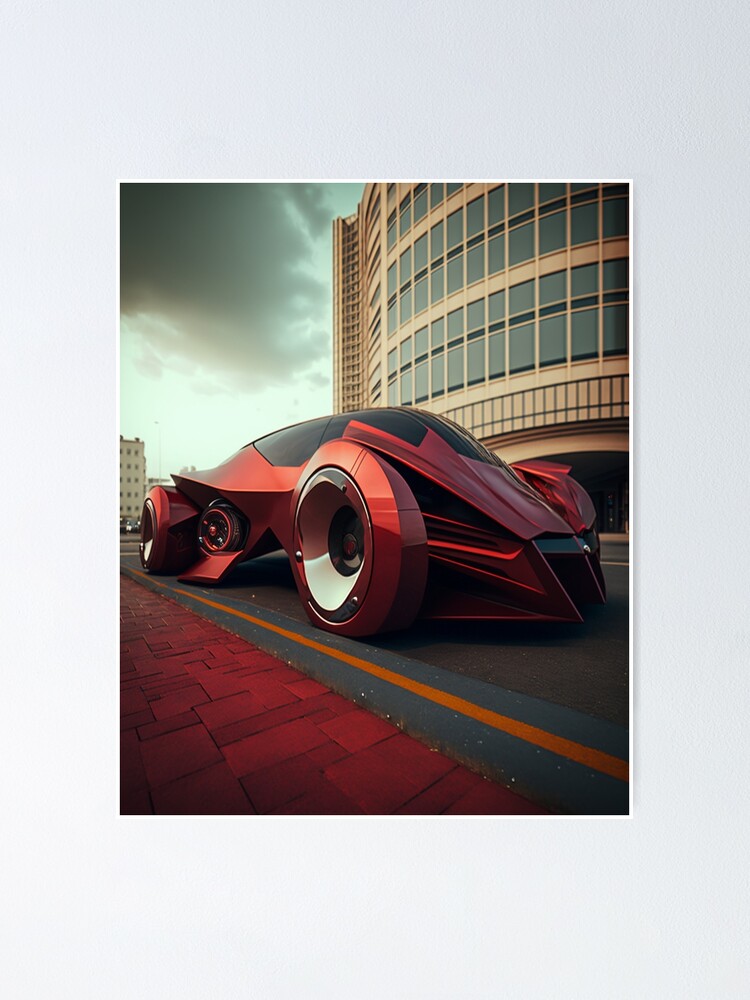This image showcases a highly futuristic car, reminiscent of something from a hundred years into the future. The sleek vehicle, painted in a striking reddish-orange hue, is parked on a street, drawing immediate attention with its sharp, low-profile design. The car's domed roof, which seamlessly integrates with its windshield and side windows, is constructed of dark smoked glass, giving it a unified, streamlined appearance. 

The car boasts enormous wheels that nearly reach two-thirds the height of the vehicle. These wheels are uniquely covered with red and chrome steel shields, concealing the traditional rubber tires. The car's sharp nose slopes down to a point only 2 to 3 inches above the road surface.

Jet-inspired design elements are evident, especially in the cockpit-like driver’s seat that appears to accommodate only one person. On the side, a circular feature resembling a jet propeller adds to the vehicle's futuristic aesthetic. This circular object attaches to the side and forms a distinct V-shape up towards the door.

The surrounding environment complements the car's modern vibe. It is parked on a road marked by a yellow boundary line, separating it from a sidewalk paved with bright red bricks. The background features a prominently rounded building with a glass façade, alongside a conventional rectangular high-rise building, enhancing the urban setting.